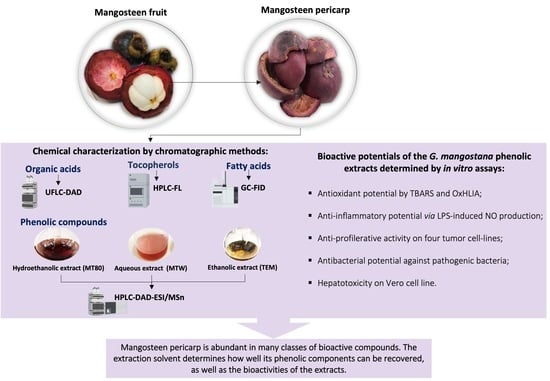The image, set against a plain white background, features a detailed chart about the mangosteen fruit and its pericarp. At the top, within gray circles, are two pictures: one of the mangosteen fruit, a deep purple, plum-shaped fruit with a white section in the center, labeled "Mangosteen Fruit," and next to it, a plate labeled "Mangosteen Pericarp," likely showing the outer rind of the fruit. Below these, a purple-bordered section contains extensive text detailing the chemical characterization of mangosteen using chromatographic methods. The text mentions the analysis of organic acids, tocopherols, fatty acids, and various bioactive potentials, including antioxidant, anti-inflammatory, antiproliferative, antibacterial activities, and hepatotoxicity, determined by in vitro assays. An arrow from this section points downward to another lilac-colored box explaining that the mangosteen pericarp contains numerous bioactive compounds, with the effectiveness of extraction depending on the solvent used, thereby impacting the functionality and recovery of its phenolic components.